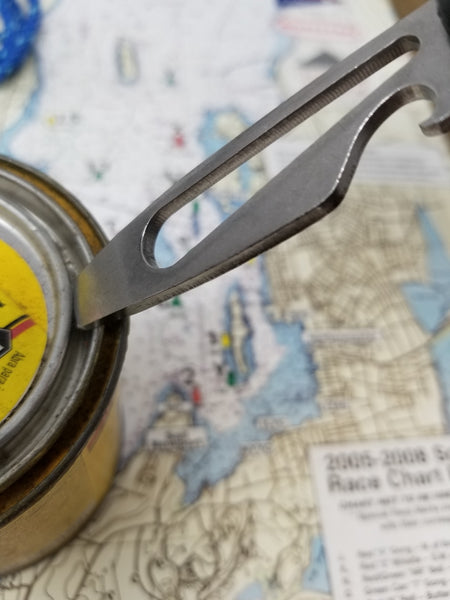This horizontally aligned photograph features a blurred and somewhat faded map as its background, variously showcasing land and sea formations. The top portion of the map is filled with wavy lines delineating larger land areas, divided by black lines, possibly denoting countries or counties. The land on the map is primarily light yellow, with some sections thickening into two rectangular shapes, one vertical and one horizontal, near another body of water with a square-shaped land protrusion. The map includes red, green, and yellow dots, possibly indicating specific towns. In the foreground, there's a prominent metal object that looks like an old-fashioned can opener, with a partially visible round yellow disc at its base, flanked by black and red stripes. The yellow disc, slightly skewed towards the inner circle's bottom, is bordered by several concentric metal rings or discs. Additionally, there is a blue plastic object located in the upper left corner. A label in the right-hand corner of the map reads "2006-2008" with a partially legible inscription beneath it. A long, slightly curved silver metal piece, possibly another part of the can opener or a knife-like tool, extends diagonally across the image, with a central notch cut out allowing the map to remain visible through its length.